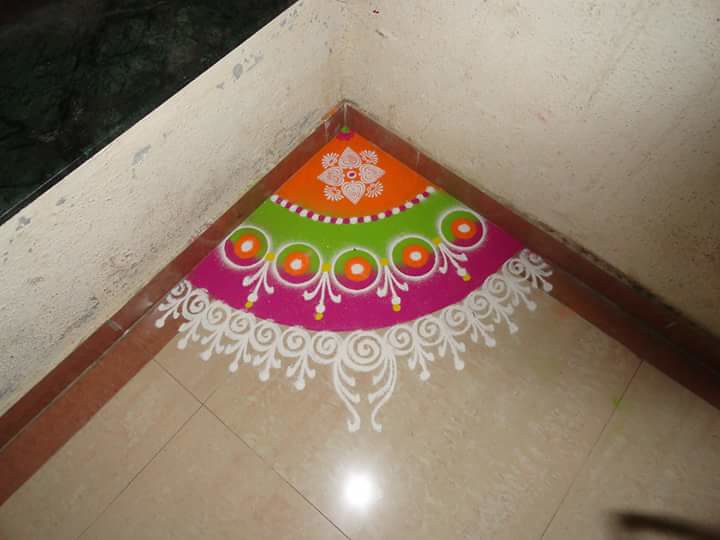This photograph captures the corner of a room with a distinctive decorative feature. The room features a beige, tiled floor and white walls with visible dings and scraped paint. A wooden baseboard runs along the walls, enhancing the room's modest design. The focal point of the image is a multicolored, lacy doily that has been meticulously placed to fit snugly in the corner. The doily, resembling an open fan with its pointed end in the corner, exhibits a vibrant pattern, starting with a floral-decorated orange segment closest to the wall. Moving outward, the design transitions through green with circular decorations, then purple, and is finally framed with a frilly, white edge. The room appears somewhat aged and simple, suggesting an attempt to add a touch of beauty and character through this colorful fabric ornament.